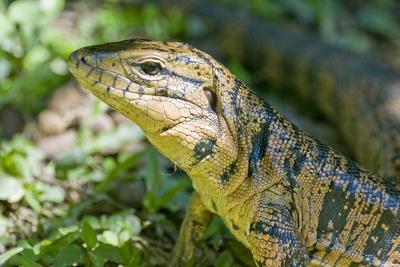This close-up photograph showcases a lizard, possibly a gecko, in its natural outdoor habitat. The lizard is predominantly a blend of light olive and yellowish light green hues with notable uneven blue stripe markings. The creature features a thick body with a fairly blunt head, tapering to an obtusely pointed nose. Its back displays slightly darker olive shades, interspersed with forest green stripes and patchy neon blue lines running horizontally in two sections. The lizard is oriented leftwards, revealing large, black eyes and dark green facial spots. The background, consisting of green foliage, twigs, and some dirt, is blurred, with varying light conditions—darker towards the upper right and illuminated from the bottom left to upper left by sunlight. The lizard's tail is faintly visible, extending over its head area and blending into the backdrop. Overall, the detailed coloration and natural setting provide a vivid and engaging depiction of this reptile.